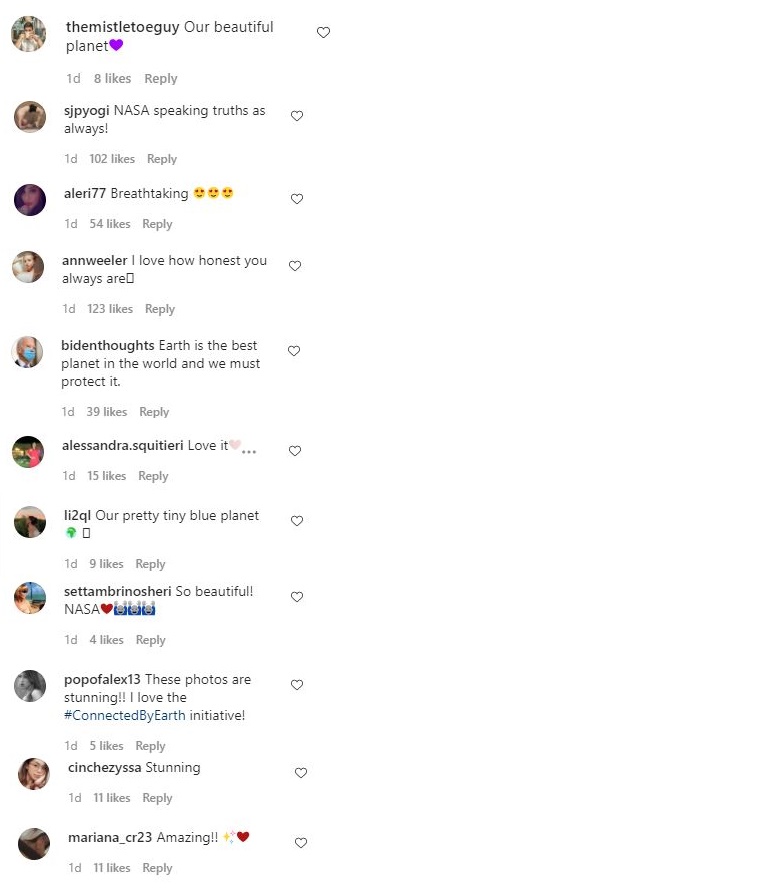This is a screenshot of Instagram comments. Each comment features an avatar to the left and a grey outlined, unfilled heart on the right. 

1. The first comment is from user "missiletypeguy" who says, "Our beautiful planet ❤️" One day ago, 8 likes received.
2. The second comment is from user "SJP_Yogi" who mentions, "NASA speaks the truth, as always." One day ago, 12 likes received.
3. The third comment is from user "Laurie77" stating, "Breathtaking 😍😍😍" One day ago, 54 likes received.
4. The fourth comment is from user "Anna_Wheeler" expressing, "I love how honest you always are." One day ago, 123 likes received.
5. The fifth comment is from user "Biden" who says, "Earth is the best planet in the world. We are the most protected." One day ago, 39 likes received.
6. The next comment from user "Alessandria.squirt" reads, "Theory love it ❤️..." One day ago, 15 likes received.
7. The next comment is from user "LITQL" stating, "Our pretty tiny blue planet 🌍." One day ago, 9 likes received.
8. The next comment from user "Sam" says, "We are most sure you're so beautiful NASA. ❤️ 🙌🙌🙌." One day ago, 4 likes received.
9. The next comment is from user "Papa_Valence13" mentioning, "These photos are stunning. I love the #ConnectByEarth initiative." One day ago, 5 likes received.
10. The next comment is from user "St.Shazia" who states, "Stunning." One day ago, 11 likes received.
11. The last comment is from user "DiscourseTheArt" simply observing, "Amazing stories ❤️." One day ago, 11 likes received.